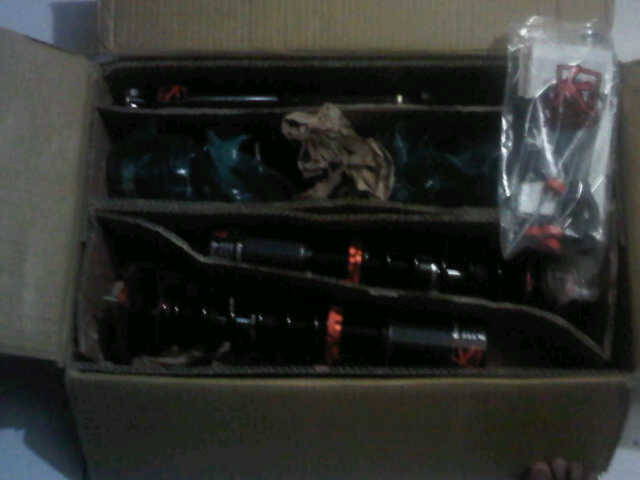A blurry, low-resolution, color landscape image shows a bird’s eye view of an open cardboard box being held open by human hands and feet, with visible toes and fingertips in the corners. Inside the box, context is cluttered but consists of various sections separated by dark brown cardboard dividers. The contents, mostly black with touches of orange and teal, and silvery metal at the top, suggest a collection of tools or equipment, possibly requiring assembly. A plastic bag with black and red contents and a white paper protrudes from the right side, and a crumpled piece of brown paper sits towards the top middle of the box. Overall, the poorly taken photograph attempts to capture the disorganized interior of the box.